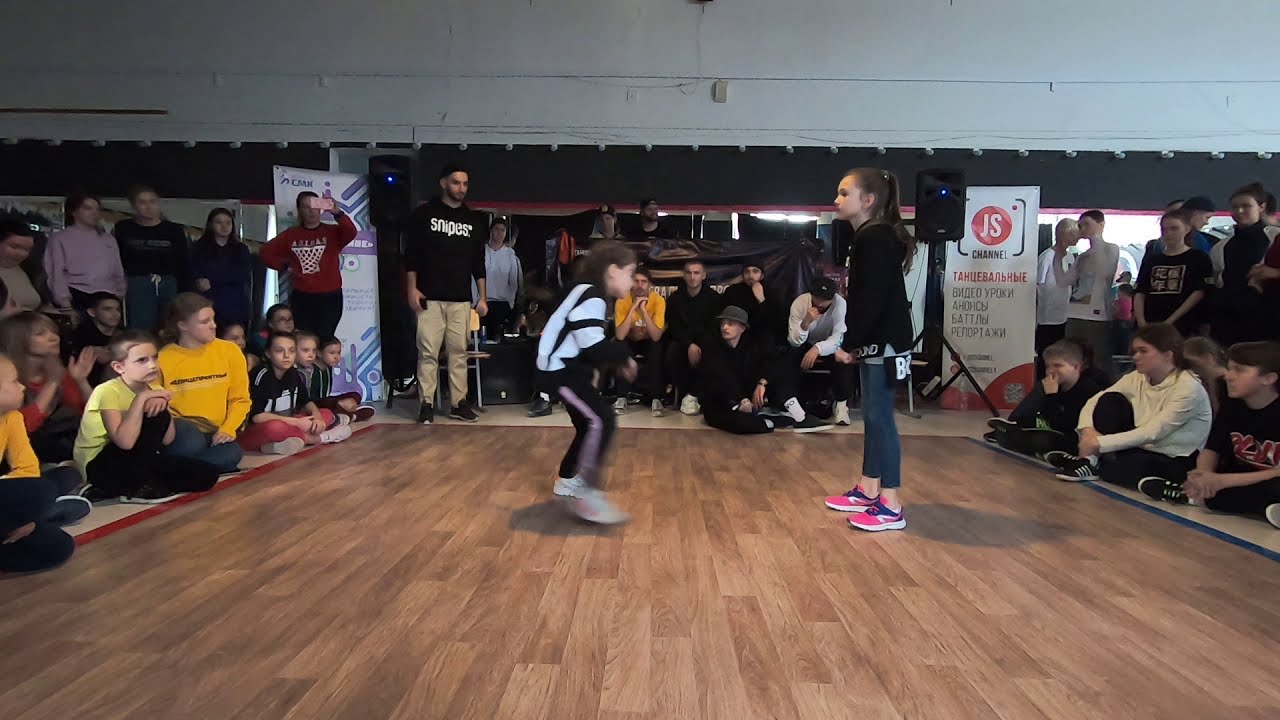In this dynamic indoor scene, two young girls appear to be participating in a dance-off on a polished wooden floor. The girl on the left, slightly blurred due to motion, wears a blue and black striped top with black pants and white sneakers, suggesting she is mid-dance. The girl on the right, standing still and watching her competitor, is dressed in a black top, jeans, and pink sneakers. They are surrounded by an audience comprised of both youth and adults, seated or kneeling on the floor around the dance area, which is bordered by thin red and blue lines. Visible in the background is a large banner or sign, partially readable with the letters "JS Channel" and additional text in what appears to be Russian. Another man in a black "Snipes" t-shirt and a woman in a red long-sleeved shirt with a basketball net design are also part of the audience, adding further details to the lively and engaging atmosphere of this indoor event, likely taking place in a gym during daylight hours, as suggested by the external lighting visible through some doors in the background.